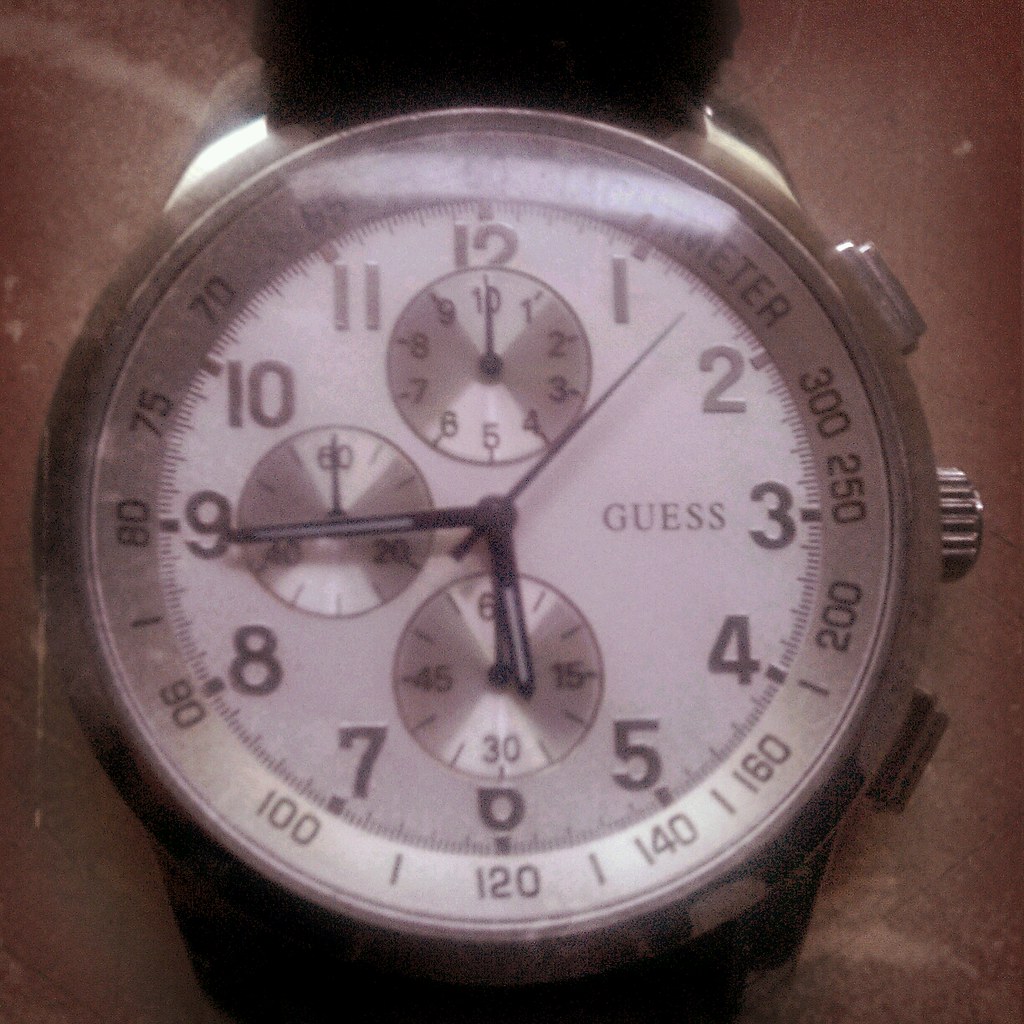A detailed close-up photograph displays a stylish wristwatch with a slight glare over the upper portion. The image features a partial view of the black band at both ends, which is somewhat cut off. The watch case is silver, showcasing a round, polished bezel. On the right side, the watch possesses two buttons and a crown, all crafted in matching silver. The watch face is white and prominently features the brand name "GUESS" in bold black lettering at the top. Traditional 1 to 12 numerals encircle the dial, marking the hours. The time is set at 5:45, indicated by black hands with white stripes. Within the main dial are three sub-dials: one for a 10-unit increment, one denoting 20, 40, and 60, and another displaying 50, 30, 45, and 60. Surrounding the watch face is a tachymeter scale, ranging from 60 to 300. The intricate details and sophisticated design elements are beautifully captured in this image.